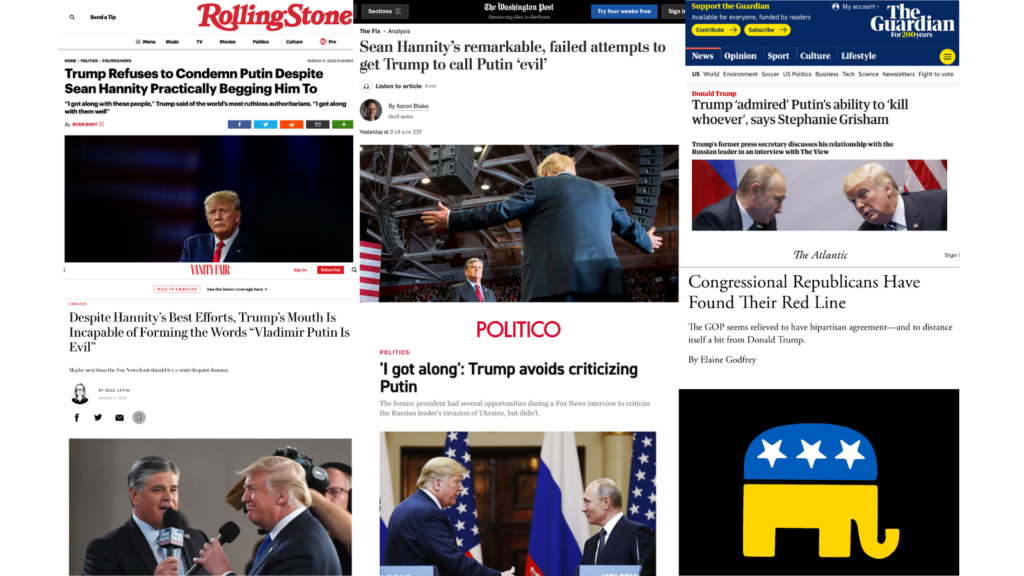This rectangular image is a collage, integrating three distinct sections seamlessly to form a comprehensive, horizontally-aligned visual narrative. 

On the far left, the visual features a prominent "Rolling Stones" logo in bold red text. Below the logo, there's a striking headline that reads, "Trump refuses to condemn Putin despite Sean Hannity practically begging him to." The main visual within this panel displays an image of Donald Trump set against a dark, bluish-black backdrop. Beneath the image, a caption clarifies: "Despite Hannity's best efforts, Trump's mouth is incapable of forming the words 'Vladimir Putin is evil.'"

The central section showcases a headline from The Washington Post, emblazoned at the top. The headline asserts, "Sean Hannity's remarkable failed attempts to get Trump to call Putin evil." Beneath this, another title from Politico states, "I got along: Trump avoids criticizing Putin," with images of both Trump and Putin included within the panel.

Finally, the rightmost section starts with a headline from The Guardian, which proclaims, "Trump admired Putin's ability to kill, whoever says Stephanie Grisham." Lower on this panel, a subheading notes, "Congressional Republicans have found their red line." Below this text, there's an illustrative graphic of an elephant—the symbol of the Republican Party—featuring a blue top with white stars and a yellowish lower body.

The amalgamation of these headlines and images in a single composite image delivers a compelling, visual commentary on Trump's relationship with Putin and the ensuing political discourse.